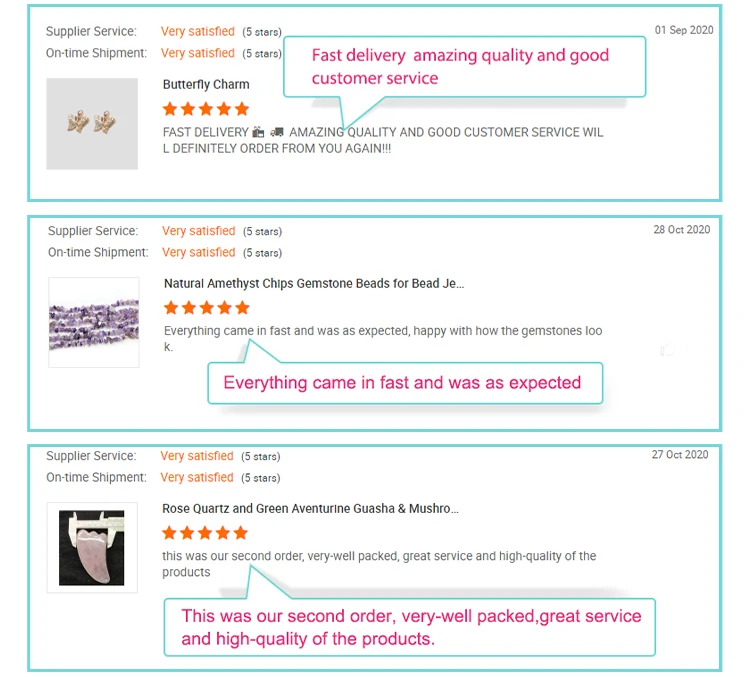A photograph showcases three detailed screenshots of customer reviews, neatly outlined in a light teal green color. Each screenshot highlights the exceptional service and quality provided by the supplier.

The first review, dated September 1st, 2020, features an image of a butterfly charm accompanied by two gold charms. The review displays five yellow stars for both supplier service and on-time shipment, each marked as "Very satisfied." Additionally, a prominent pink pop-up box overlays the review, boldly stating "Fast delivery, amazing quality, and good customer service," which is reiterated in black font below.

The second review, dated October 28th, 2020, includes a picture of natural amethyst gemstone beads. This review similarly awards five stars for both supplier service and on-time shipment, describing them as "Very satisfied." A pink box accentuates the feedback with the message: "Everything came in fast and was as expected."

Lastly, the third review, dated October 27th, 2020, showcases a set of gua sha tools made from rose quartz and green aventurine. Consistent with the previous reviews, this one also provides a five-star rating for the supplier service and on-time shipment, emphasizing total satisfaction with both.

Each review collectively underscores the prompt delivery, high quality, and excellent customer service consistently provided by the supplier.